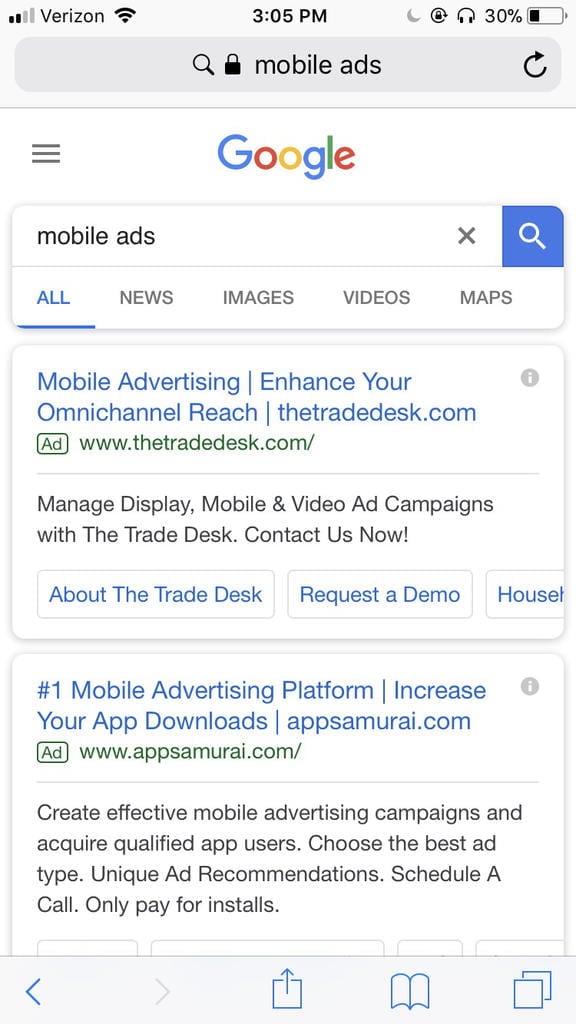This mobile device screenshot captures a Google search on "mobile ads," reflective of a typical user interface. In the upper left corner, the cell signal indicator shows Verizon as the carrier, accompanied by a Wi-Fi symbol. Centrally positioned at the top, the time reads 3:05 p.m., flanked on the right by a headphone icon, the auto-rotate lock symbol, and a battery indicator at 30%. 

The user's search term "mobile ads" is entered in the web browser bar beneath these status indicators. The familiar Google logo appears at the top of the search results, followed by tabs for "All," "News," "Images," "Videos," and "Maps" searches. The initial search results display paid advertisements. The first ad, from thetradedesk.com, highlights "Mobile advertising: Enhance your omnichannel reach." Directly below, another ad from appsamurai.com promotes the "Number one mobile advertising platform" with a focus on increasing app downloads. Both advertisements are marked with grey information circles on their right side, indicating their ad status.